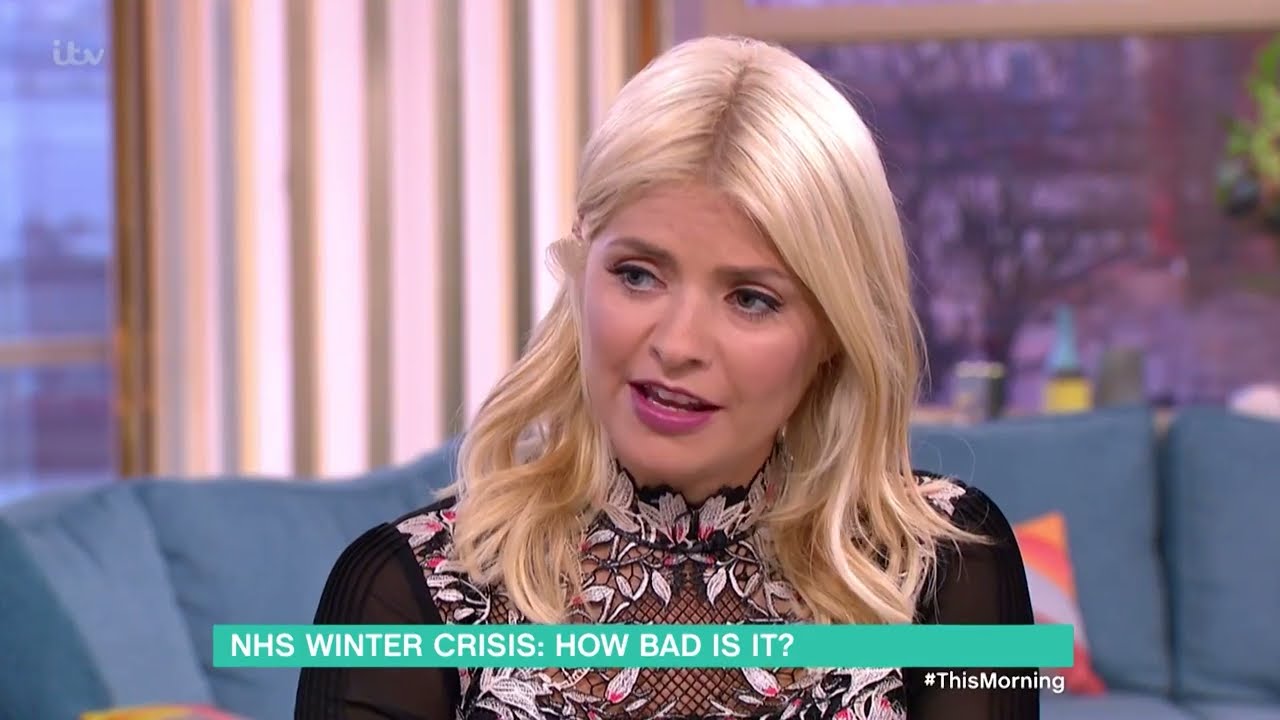The image captures a screenshot from a morning talk show set in a living room-like environment. The set includes a teal sectional couch adorned with pillows in vibrant colors such as orange, red, pink, and white stripes. The background features windows with white curtains that overlook trees, contributing to a lifelike yet artificial studio ambiance. In the scene, a blonde woman, likely in her 40s, is the guest. She has light blonde hair parted in the middle, with her hair tucked behind her right ear, and is wearing magenta lipstick along with mascara and eyeshadow. Her black, high-neck blouse features sheer, gauzy sleeves and floral appliqués in white and pink. She sits slightly turned, looking towards the left of the camera. At the bottom of the image, a teal-colored rectangle with white capital letters displays the caption “NHS winter crisis: How bad is it?” followed by the hashtag “#ThisMorning.” An ITV logo is visible on the upper left side of the image.